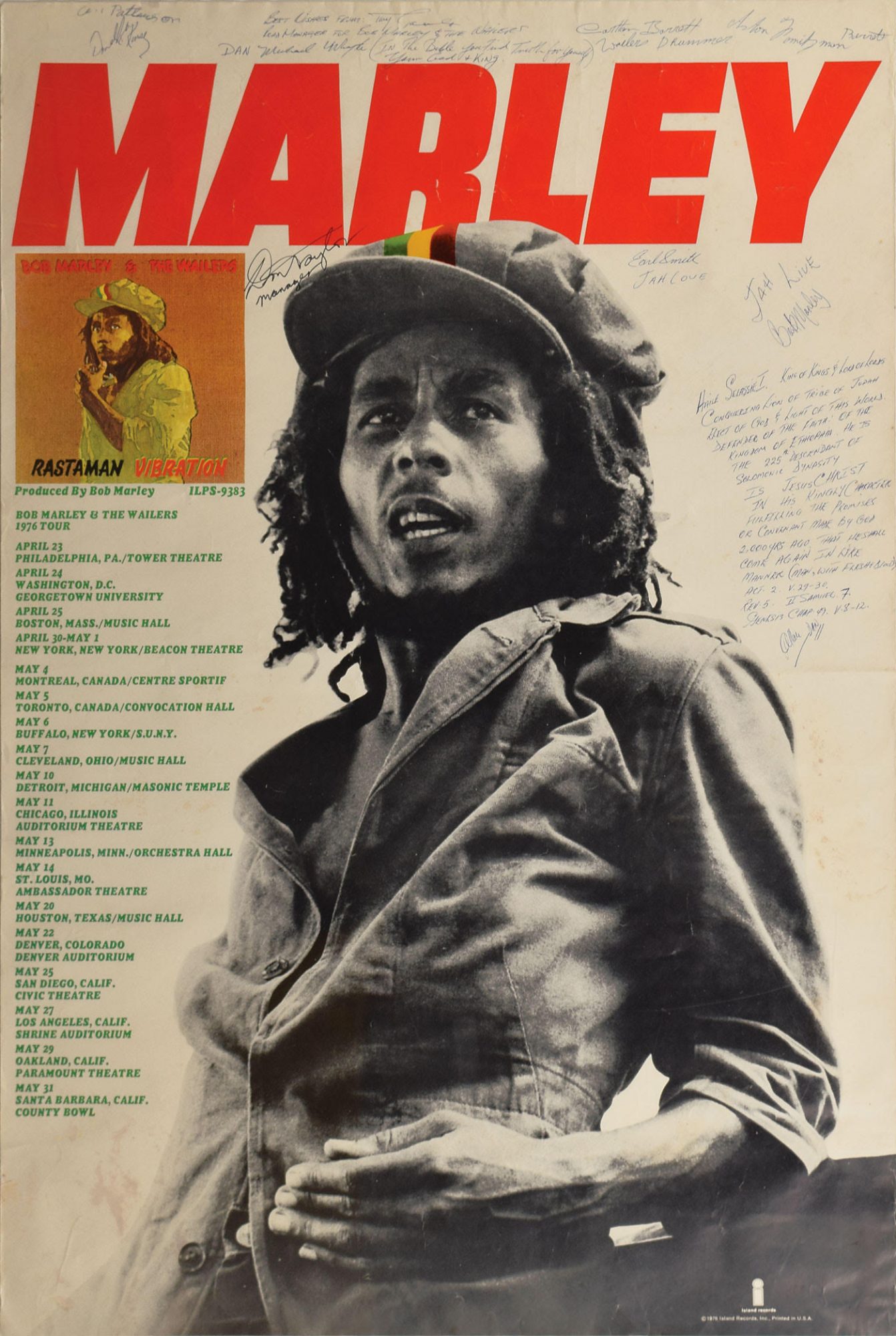This detailed image is an aged tour poster for Bob Marley. The poster's paper has yellowed over time, giving it a vintage look. At the top, "MARLEY" is emblazoned in big, bold capital red letters. Just below this title, on the left side, is a small square painting of Bob Marley, identifiable by his long dreadlocked hair, mustache, and beard. In this artwork, Marley is depicted with his left hand raised to his face and wearing a light green cap adorned with three horizontal stripes in green, white, and red down the center. His light green shirt with long sleeves is rolled up to his elbows. 

Following this, the phrase "Rastaman Vibration" appears in black text. Dominating the center of the poster is a black and white photograph of Bob Marley, showcasing him in a casual pose as if conversing with someone. He sports his iconic hat, which in this photograph features colored stripes of green, yellow, and red. Marley's shirt is a button-down, open with most buttons undone. 

Adjacent to the photograph on the left margin is a list of tour dates and locations, written in green text. This list details Bob Marley's 1976 tour with locations spanning multiple cities from Philadelphia, PA, to Santa Barbara, CA, complete with dates and venues such as the Tower Theater and the Beacon Theater. Scattered across the remaining open spaces of the poster are small, handwritten notes or signatures in mostly blue ink, adding a personal touch. The authenticity of the content is further solidified by the production credit, "Produced by Bob Marley," mentioned within the textual details.